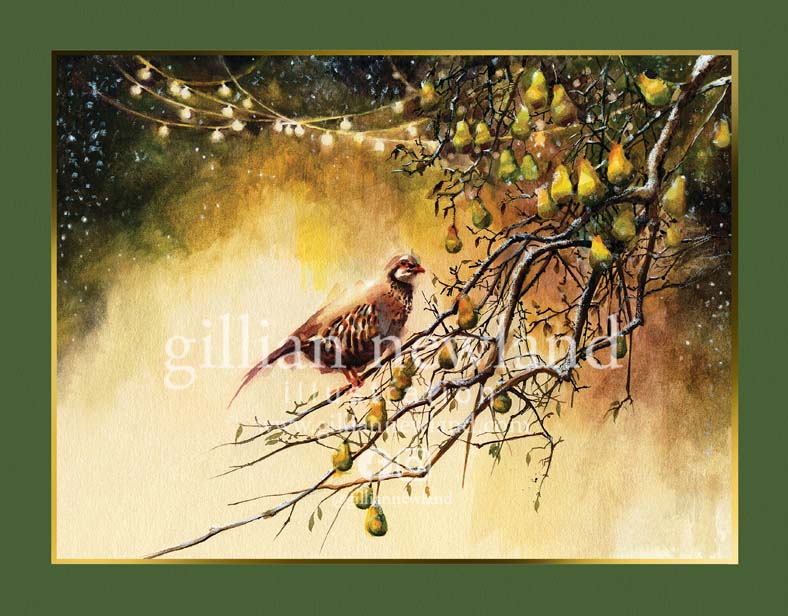This rectangular painting, measuring approximately six inches wide by four inches high, is bordered by a dark green frame about a quarter to a half inch thick, which is further accentuated by an inner gold border about an eighth of an inch thick. In the painting's center, a partridge bird perches on a slender branch of a tree that extends diagonally from the upper right corner toward the lower left, just shy of the painting's edge. The bird, facing right, showcases predominantly brown feathers with white patches, a distinctive red beak, and a tiny tuft of white feathers on its forehead, complemented by a white spot beneath its chin outlined in black. The branch is laden with green and yellow pears, adding vibrant detail. Illuminating the upper portion of the painting, strings of small white lights hang from the tree's branches. The background transitions from a cream color at the bottom to a rich blend of green, orange, and yellow towards the top. The painting features a watermark across the middle which reads "Jillian Newland," although finer text beneath it remains indecipherable.